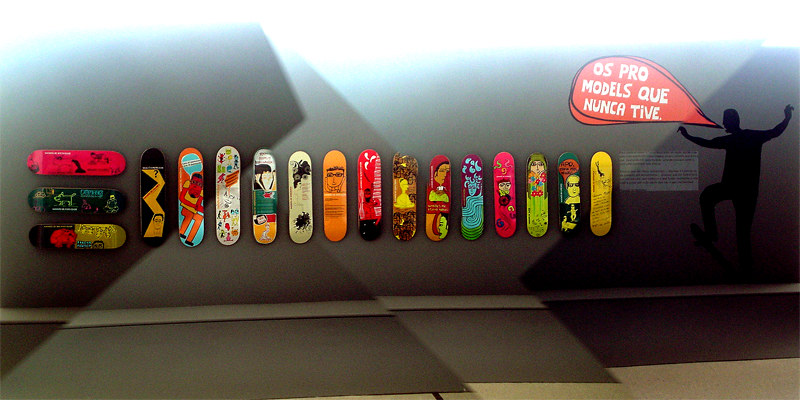The image depicts a stylish graphic design showcasing a collection of skateboards arranged on a wall. There are 15 skateboards in total, featuring vibrant artwork that includes portraits and mosaic-like designs with shades of orange, pink, red, and yellow. Along the left side, three skateboards are positioned horizontally, while the remaining 12 are arranged vertically next to them. In the upper right corner, a black silhouette of a man with outstretched arms is seen, accompanied by a large red speech bubble with the Portuguese phrase "Os pro models che nunca tive." The background features a gray and white palette, adding a contrasting backdrop to the colorful skateboards and the striking black silhouette.